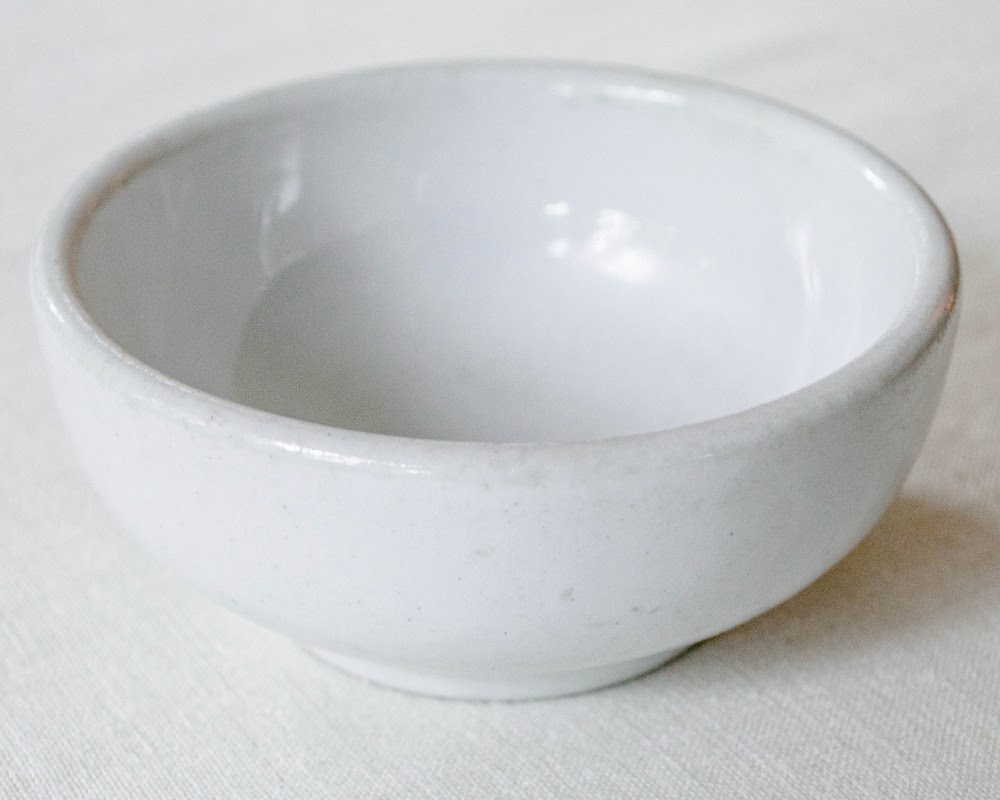This image features a white ceramic bowl, possibly handmade, positioned on a pristine white linen tablecloth. The tablecloth exhibits neat, pressed stitching running both vertically and horizontally, adding a subtle textural element to the scene. The bowl itself is shallow, small, and entirely white save for some shadowing and a hint of brown around the top, likely a result of professional lighting. The light glints off the bowl's surface, suggesting an artful presentation reminiscent of a museum or gallery display. The composition is simple and monochromatic, with intricate reflections and light patterns both within the bowl and on the tablecloth.